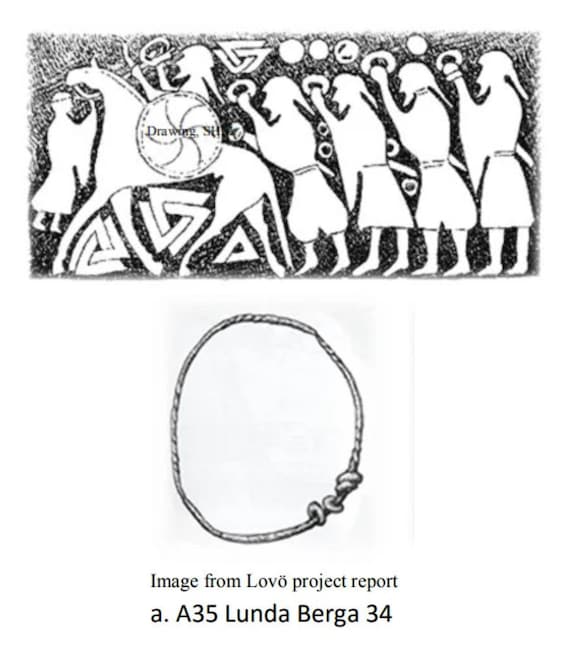The image comprises two photographs against a white background. The top photograph features a medieval-style illustration depicting a scene with a dark-to-light gradient backdrop and cross-hatching details. Central to the illustration is a stylized horse with a rider who appears to be a soldier holding a shield and an indeterminate instrument, riding to the left. In the scene, there are four male figures, possibly soldiers, standing in a row behind the horse, each equipped with swords at their waists and holding circular objects, possibly tambourines. Additionally, there is a monk or priest figure in front of the horse. Surrounding these figures are Viking-era symbols, including intertwined triangles or Valknuts. The soldiers are dressed in kilts or shorts and boots, adding to the medieval atmosphere. Below this illustration, the second photograph displays a silver bracelet with an abraded surface, an oblong-oval shape, and knot details. Beneath the bracelet is a caption reading, "Image from Lovo project report. A.A35 Lundeberga 34," possibly indicating the source and age of the image, suggesting it could be ancient or medieval in origin.